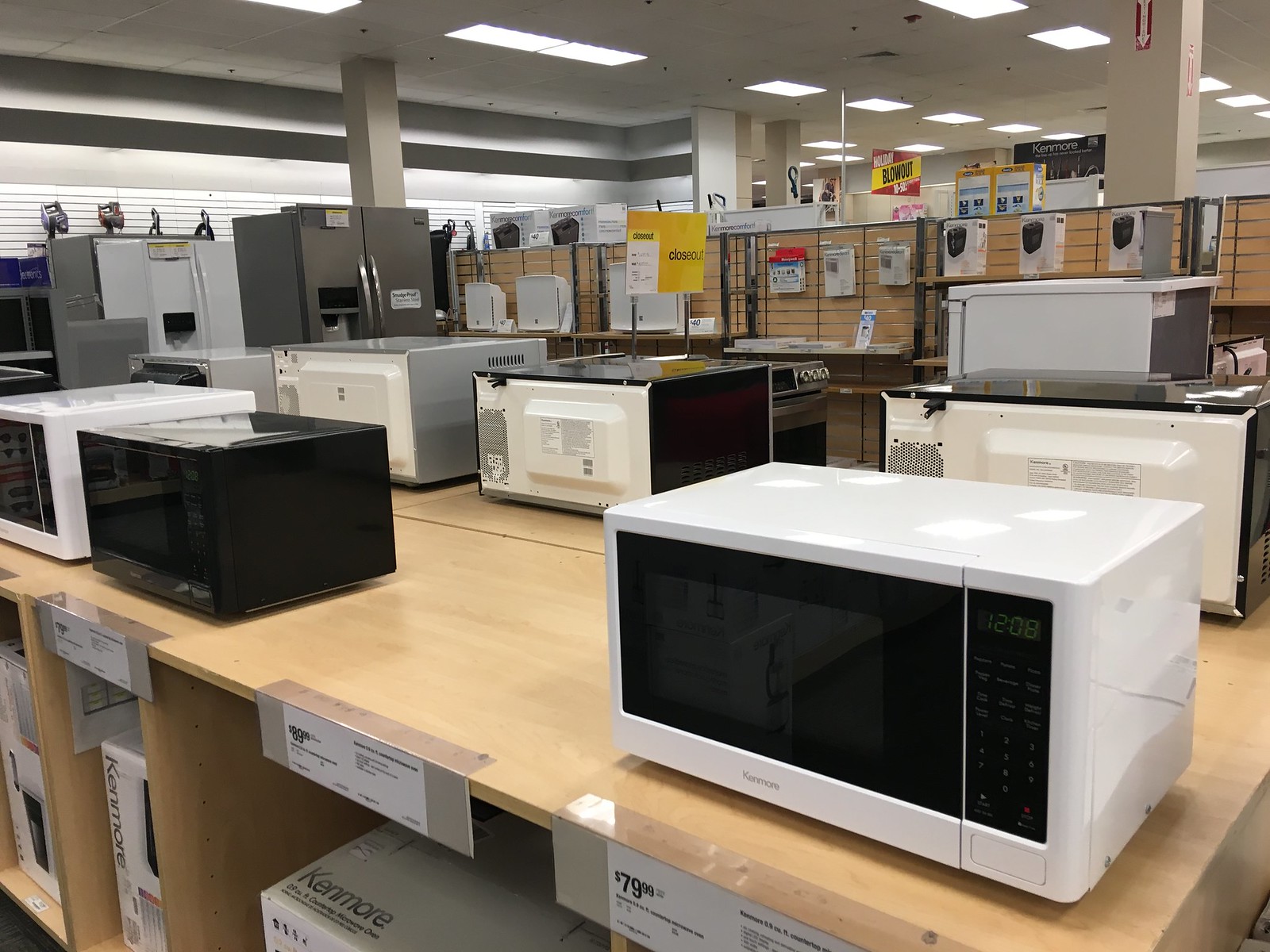The image is a color photograph taken inside a commercial electronics store or appliance outlet. In the foreground, birch-colored benches slightly diagonal from right to left display various microwave models. Some microwave models have sold out, indicated by empty spaces and plastic holders with pricing labels along the front lip of the surface. Beneath these benches, boxes containing the microwave models are stacked, ready for customers to pick up and purchase.

Behind the microwaves, additional rows of appliances can be seen, including the backs of more microwaves on a mirrored table setup. To the left of the image, additional shelves hold various other items for sale. In the back left corner, free-standing side-by-side refrigerators are visible, and along the left back wall, electric cooling fans are displayed. 

The ceiling is equipped with fluorescent lights, illuminating the store brightly, and grey pillars support the structure. Several signs hang from the ceiling and shelving units, advertising prices, slogans, and clearance offers in colors like red and yellow. Although specific brand names like Kenmore are mentioned, details are not clear enough to read distinctly. The overall ambiance suggests a busy, well-stocked retail environment dedicated to home appliances.